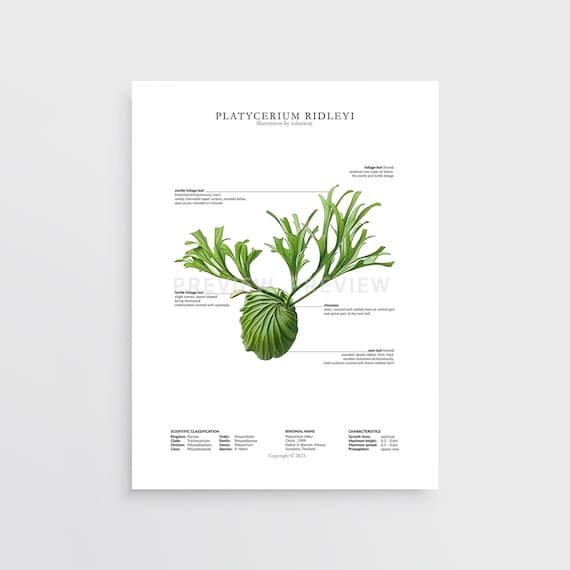The image depicts a sample template page predominantly showcasing a staghorn fern, scientifically named Platycerium ridleyi, positioned centrally against a white background. At the top of the page, the Latin name "Platycerium ridleyi" is written in all capital letters, serving as a title. Below this title, the plant is displayed with its green, dusty green, cabbage-like leaves fanning out reminiscent of stag's horns. Surrounding the plant image, there's black text intended for descriptive purposes, but it is too small and blurry to read clearly. In the middle and bottom sections of the template, additional black text is present, and a watermark reading "preview, preview" is superimposed over the page, indicating that this is a preliminary version designed to show what the final plant description layout might look like.